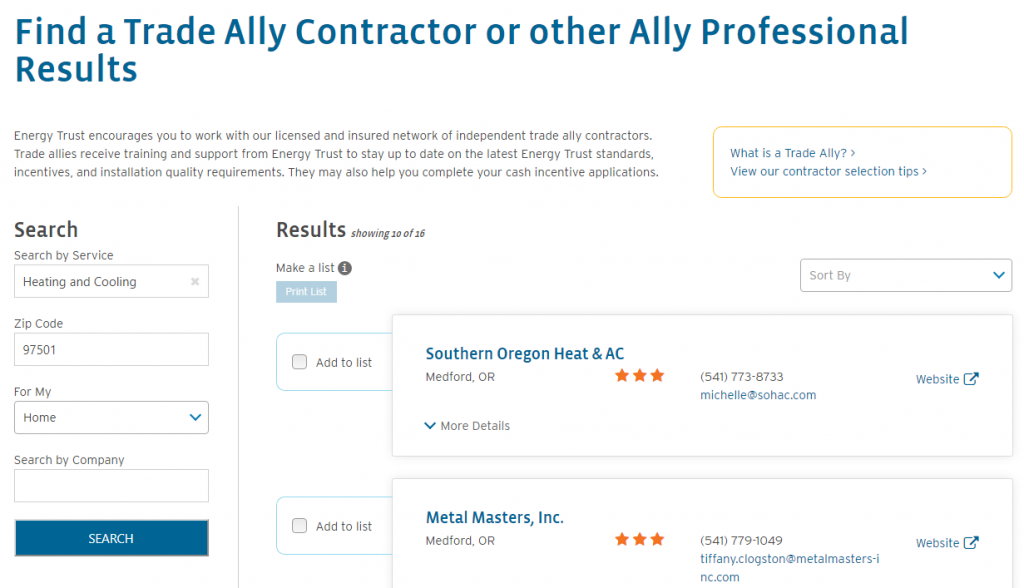This image is a detailed screenshot from a website designed to help users find trade ally contractors or other professional allies. Near the top, there is a prominent header that reads, "Find a Trade Ally Contractor or Other Ally Professional Results." Below this header, a paragraph explains that Energy Trust encourages users to work with its network of licensed and insured independent trade ally contractors. These contractors receive specialized training and support from Energy Trust to stay current with the latest standards, incentives, and installation quality requirements. They may also assist in completing cash incentive applications.

On the right side of the image, there is a rectangle outline containing two buttons labeled, "What is a Trade Ally?" and "View Our Contractor Selection Tips." To the left, a search interface includes a box labeled "Search by Service," which is pre-filled with the term "Heating and Cooling." Additional search fields include a text box for the zip code, pre-populated with '97501,' and a drop-down menu under "For My," set to 'Home.' There is also an empty text box labeled "Search by Company." Beneath these search fields, a blue search button is prominently displayed.

To the right of the search interface, two search results are listed: "Southern Oregon Heat and AC" and "Metal Masters Inc."